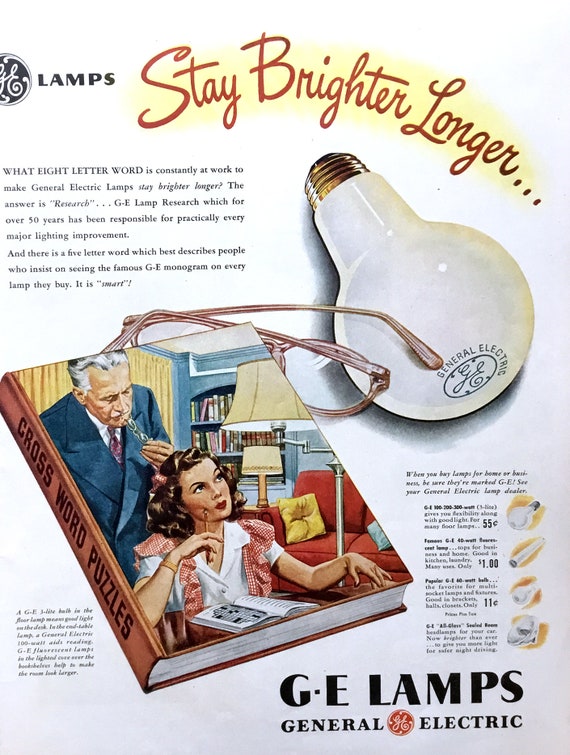This vintage advertisement poster, likely from the 1950s or 1960s, promotes General Electric (GE) lamps with the slogan “Stay Brighter Longer” prominently featured in bold red script forming a curved arc. The background is white, giving the ad a clean and classic look. At the top left corner, the iconic GE logo is displayed in red alongside the word "LAMPS" in bold black letters.

Below the title on the right side of the poster, there is an image of a standard GE light bulb, shown upside down with the screw-in portion pointing upward and the illuminated bulb downward. The General Electric logo is clearly visible on the bulb's top. To the left of the light bulb, a pair of reading glasses rests beside a book titled "Crossword Puzzles." The cover of the book features an illustration of an older man standing behind a younger woman, who is seated at a desk and appears to be working on a crossword puzzle.

A subtitle engages the viewer with a riddle related to the GE lamps, asking, “What eight-letter word is constantly at work to make General Electric lamps stay brighter longer?” The answer provided is “research,” highlighting GE's long-standing commitment to innovation in lighting technology. It further teases with another riddle, “And there is a five-letter word which best describes people who insist on seeing famous GE monogram on every lamp they buy,” with the answer being “smart.”

The bottom of the ad reiterates the brand with the phrase “GE Lamps” in prominent black capital letters, followed by “General Electric” and the familiar red GE logo. Smaller groups of text are scattered throughout, but they remain difficult to read due to their small size. Overall, this ad conveys a blend of reliability and ingenuity, characteristic of GE's marketing from mid-20th century.